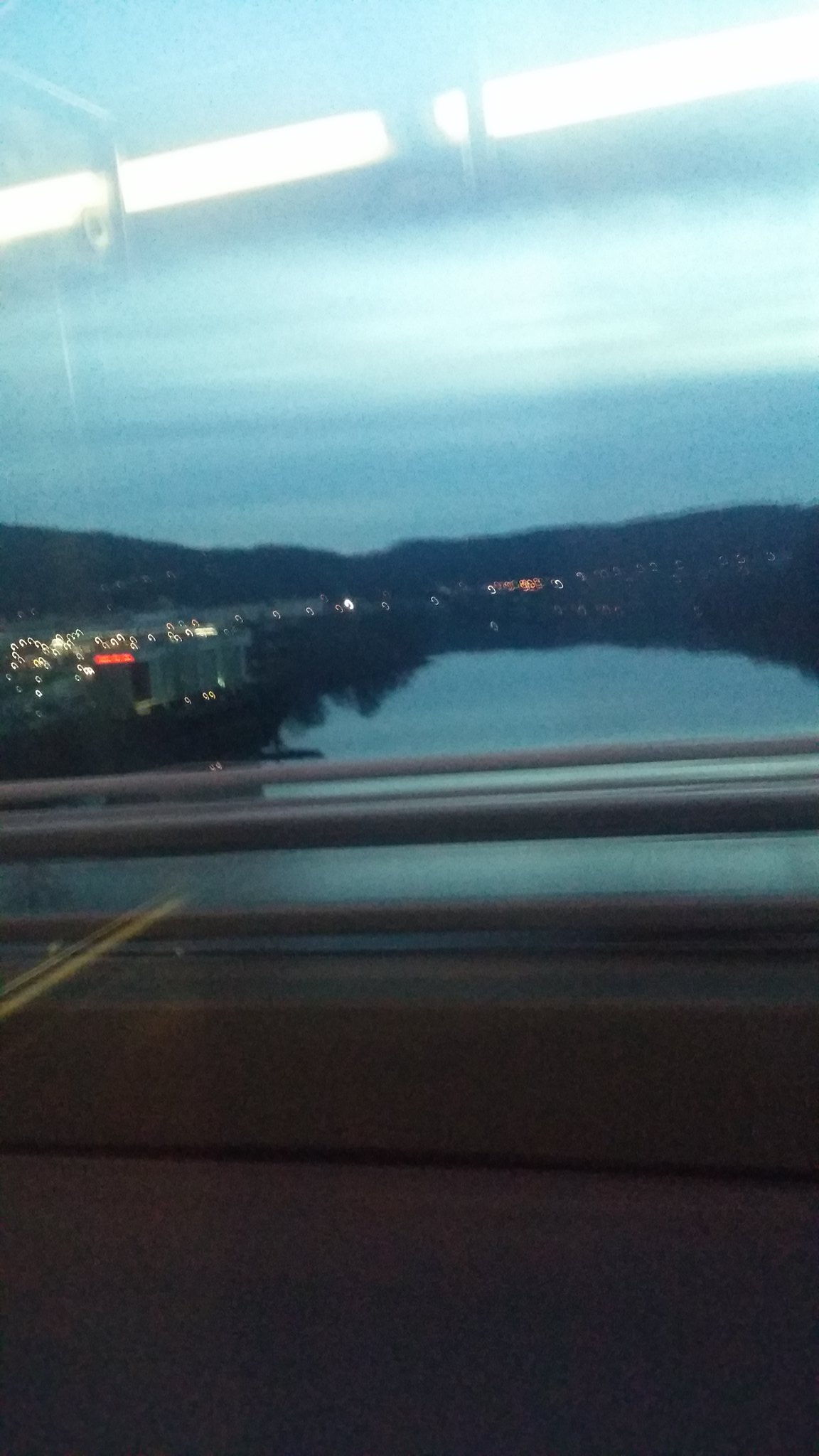A deceptive first glance suggests a bridge view, but upon closer inspection, the scene reveals an interior setting with a large picture window. In the upper left corner, a ceiling and three long white lights are visible. What initially looks like the parapet of a bridge is, in fact, a windowsill. Beyond the window, a broad river stretches across the scene. The left riverbank is heavily developed, featuring numerous buildings with illuminated windows. Among these, a red sign with white text stands out, though its message remains unreadable from this distance. The dark sky indicates it is either very early morning or nighttime.